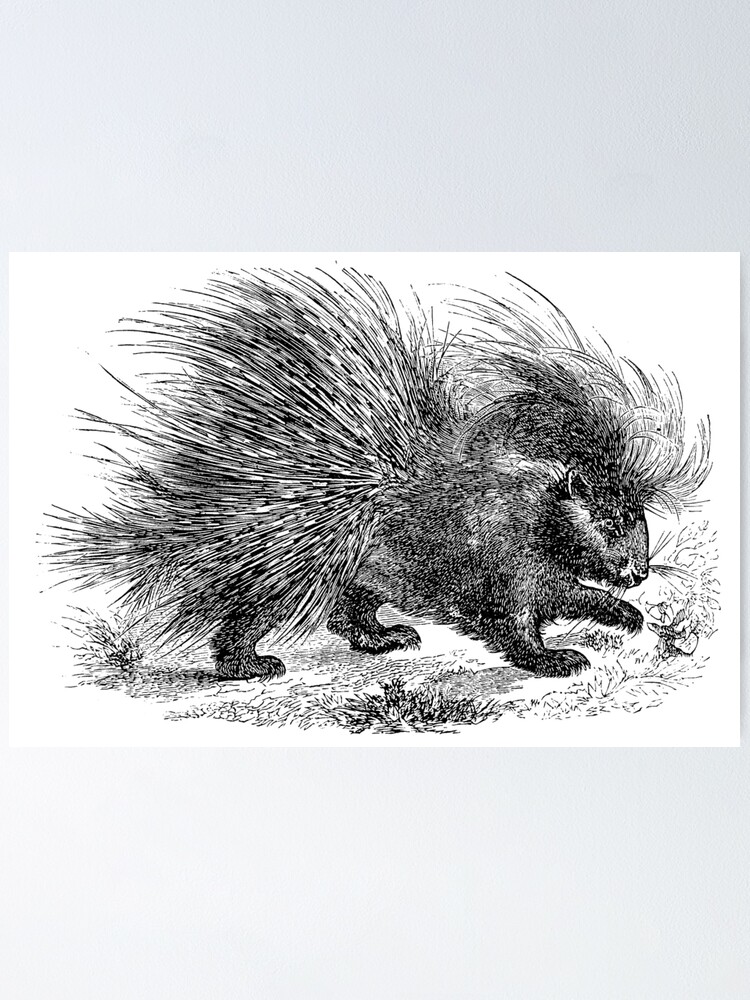This is a detailed drawing of a porcupine, rendered in what appears to be charcoal or crayon on a white sheet of paper, resembling an illustration you might find in a children's book. The artist employed a shading technique, giving the porcupine a bushy, fuzzy appearance, with its long black quills prominently standing out against the white background. The porcupine, depicted in mid-stride with one leg slightly extended, seems to be sniffing or interacting with a small object on the dry, sunny ground, possibly a piece of vegetable. The surrounding grass is drawn to appear dry, indicating a daytime setting. The porcupine has a narrow face, four legs with two front paws and two back paws, and its distinctive quills are ready to puff out defensively if needed. The overall composition suggests a scene of the porcupine exploring its environment, perhaps on a leisurely stroll through a sunlit field.